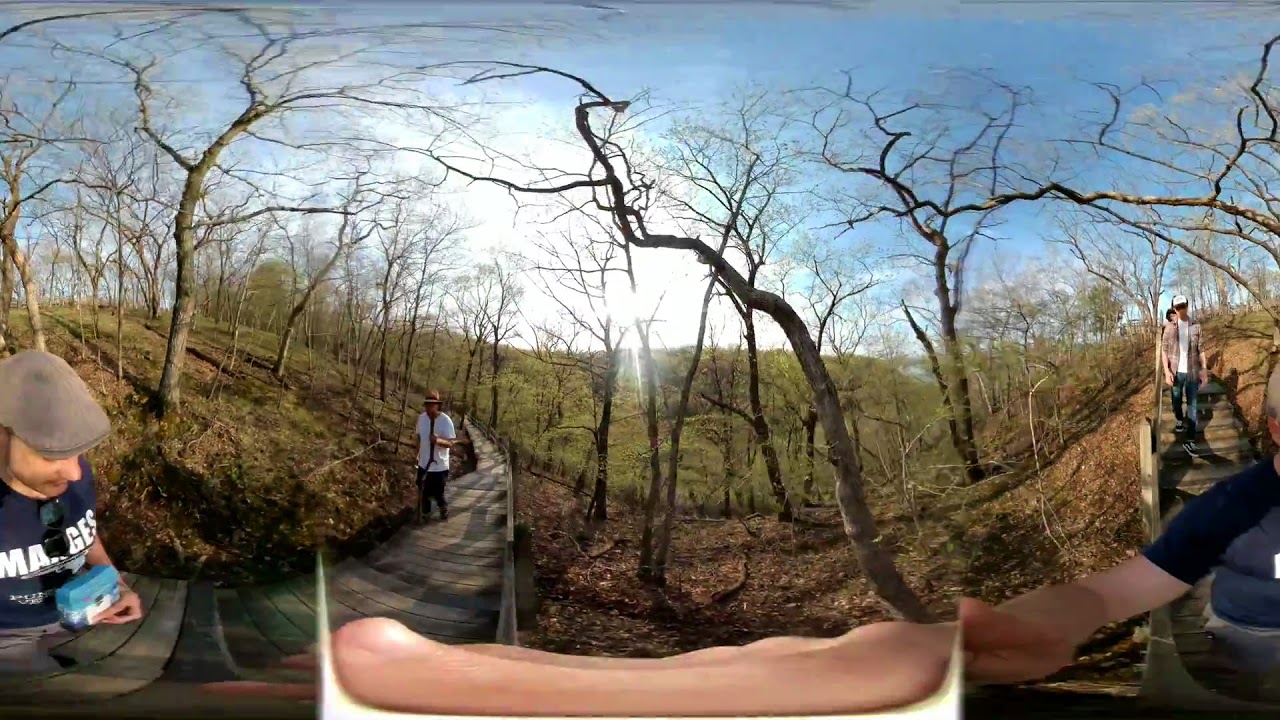In this panoramic outdoor image, a group of people is seen hiking through a scenic forest area, highlighted by a wooden walkway that meanders through the leaf-strewn ground. The season appears to be late fall, as the trees are barren of leaves, their scraggly branches resembling veins against the clear blue sky. Warm sunlight bathes the scene, casting a bright glow that emphasizes the earthy tones of orange leaves scattered on the ground and patches of greenery interspersed with dirt.

At the bottom left corner, the person holding the camera is visible, wearing a gray cap and a blue t-shirt with white text. To his right, another individual donning a straw hat and white t-shirt is captured mid-hike. Further along the pathway, a man in a white hat and flannel shirt is seen walking. The scene is framed by a gradual hill leading down to a serene valley, with pathways cutting through the sparse forest. This comfortable, nature-rich setting is bustling with hikers enjoying their day outdoors, under a clear mid-day sky speckled with a few clouds.